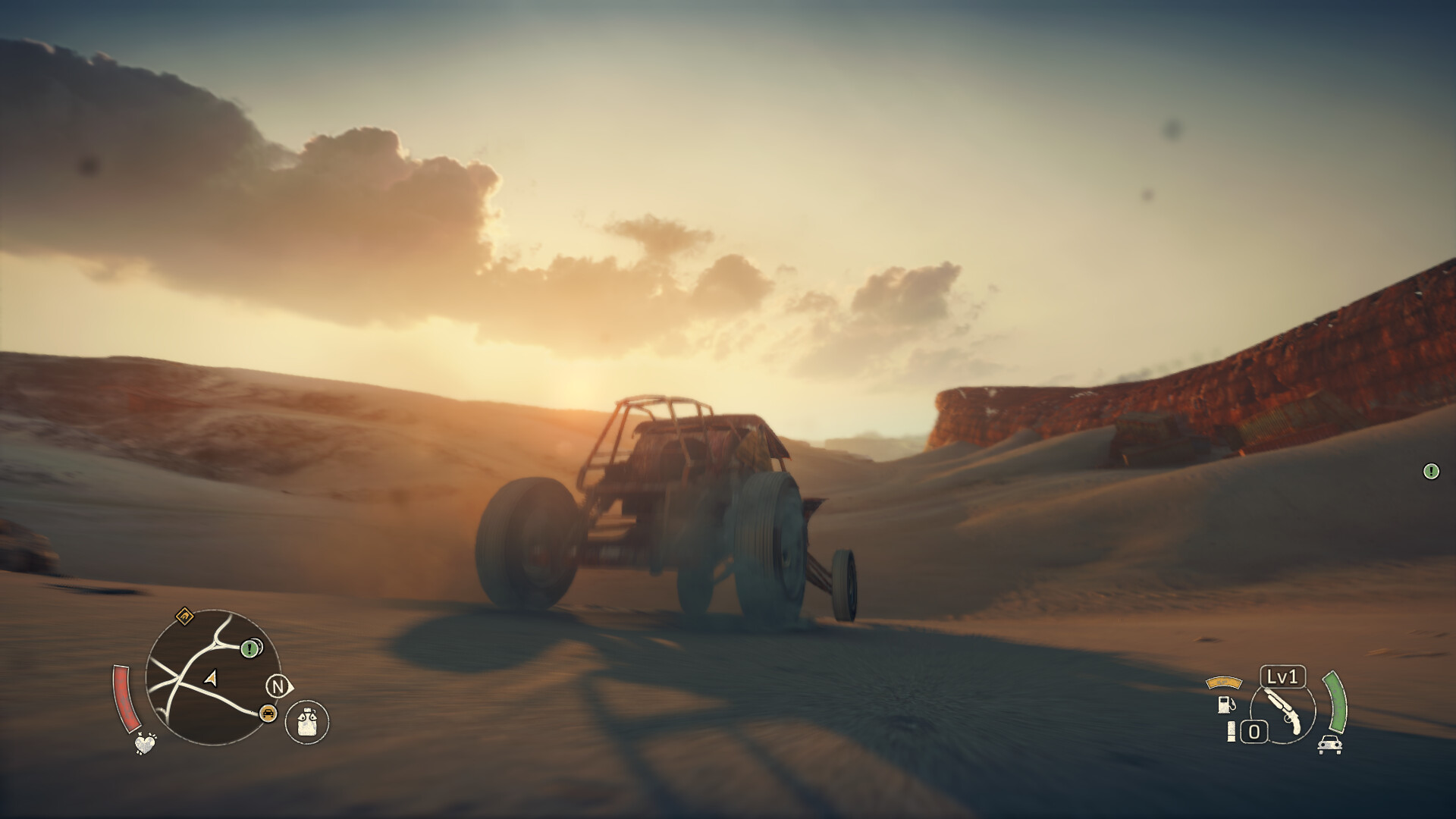This horizontal image features a rugged dune buggy positioned centrally within a vast desert landscape, surrounded by undulating sand dunes and hills. In the background, to the right, there's a striking plateau mountain standing tall against a sky sprinkled with a few fluffy clouds on the left side. The ambient light suggests either sunrise or sunset, casting a soft, muted glow that enhances the serene yet adventurous feel of the scene. 

In the bottom left corner of the image, there is a circular map with a black background and white detailing. On the bottom right, a cluster of icons can be seen. An icon of a car in white is overlaid with a green semicircle above and to the left of it. Adjacent to this icon is a circle, also on the left, with the text "LV1" positioned above it. To the left of this cluster are three distinct icons: the first is gold, the middle icon is white and shaped like a gas pump, and the third is a vertical white rectangle. To the right of the third icon, there is a small rectangle displaying the number "0" in white text.